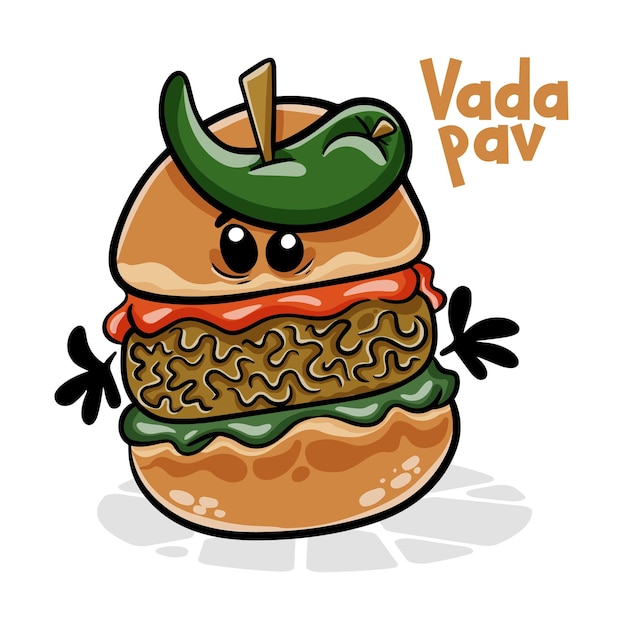The image features a cartoon illustration set against a white background, showcasing a whimsical hamburger character with anthropomorphic features. The character has a tan-colored upper bun adorned with a pair of black eyes. A toothpick pierces the top bun, skewering a green jalapeno pepper. Beneath the top bun is a layer of red, presumably ketchup, followed by a light brown patty with black squiggles. Below the patty is a green layer that could be lettuce or avocado. The bottom bun is tan with white circles, and the entire burger is standing sideways, its black-outlined hands outstretched. The character casts a gray shadow onto the white surface below it. In the upper right corner, the text "Vada Pav" is displayed in orange, written in two rows with careful spacing between the letters.